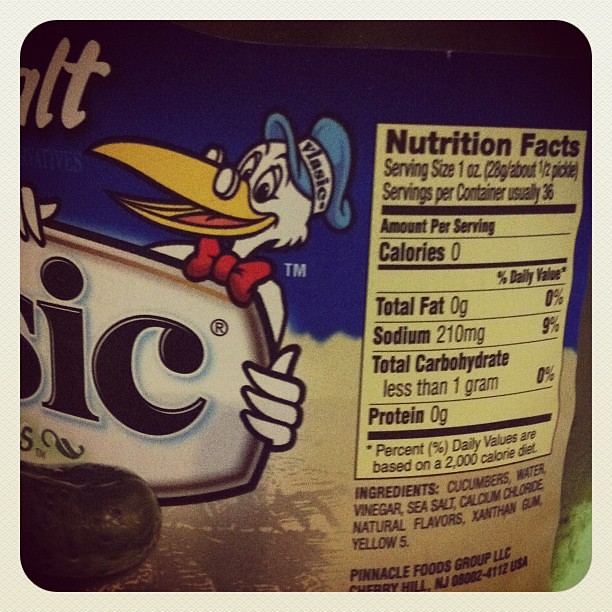This image features a close-up view of a Vlasic pickle jar label. The label is divided into two distinct sections: the front branding and the side nutrition facts panel. 

At the top of the front label, there is a royal blue background, transitioning to white at the bottom. Dominating the label is an illustration of the Vlasic mascot — a cheerful, anthropomorphic stork. The stork has a white body and is wearing a blue cap with the word "Vlasic" written on the band. He sports glasses over his eyes, has a long yellow beak with a pink tongue peeking out, and is adorned with a red bow tie. The stork is holding a sign with "Vlasic" prominently displayed in bold white letters. Below the sign, a portion of a pickle is visible.

Moving to the side of the jar, the label includes a comprehensive list of ingredients: cucumbers, water, vinegar, sea salt, calcium chloride, natural flavors, xanthan gum, and yellow 5. Above the ingredients list, the nutrition facts are detailed, providing essential dietary information.